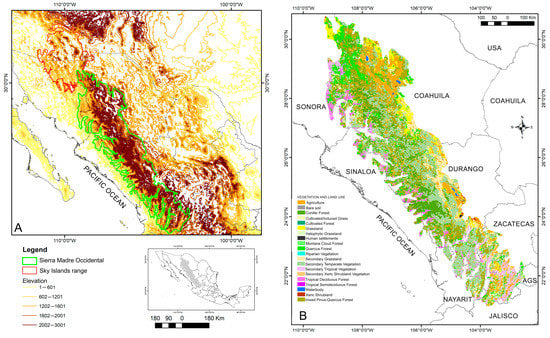The image displays two side-by-side topographic maps labeled A and B, each bordered by thin black lines and set against a white background. 

The map labeled A on the left exhibits a range of colors with red, yellow, and orange shades, depicting varying elevations of mountain ranges in Central America. Notably, the green outlines highlight the Sierra Madre Occidental, while red borders mark the Sky Island range. The map includes the Pacific Ocean, colored white, with clearly visible elevation markers and a legend detailing these features. Below map A, there is a smaller black-and-white version for additional reference.

The map labeled B on the right features more diverse colors including green, yellow, orange, and pink, marking different states and elevations. The states, including Sonora, Sinaloa, Durango, Coahuila, Zacatecas, Jalisco, and others, are bordered in white and labeled with black ink. The United States is also visible at the top right of the map. The ocean areas are white, labeled with black ink. The scale of the maps is located at the top right of the image, while the legend for map B, although small and challenging to read, is positioned at the bottom left. Both maps are detailed representations focusing on the geographical and topographical differences within Central America.